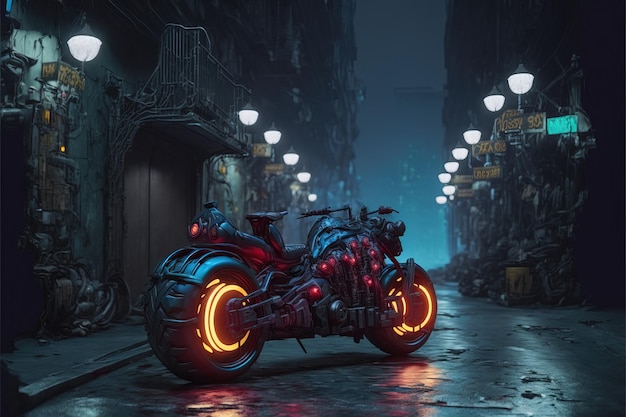The image features a detailed, artistically-rendered motorcycle set against a dark, technologically-infused cityscape that resembles a comic book or AI-generated art. This futuristic motorcycle, reminiscent of the one in the movie Tron, boasts large, glowing tires with orange-lit interiors contrasting its standard black rubber exterior. Tiny red lights or parasite-like dots accentuate the motorcycle’s sleek design. It sits prominently in the middle of a damp, reflective alleyway road at night. Surrounding the scene are run-down buildings lined with hanging lights, giving off a spooky and atmospheric vibe. The background includes a blurred view of signs and possibly a door to an apartment or retail shop, enhancing the depth and intrigue of this animated depiction.